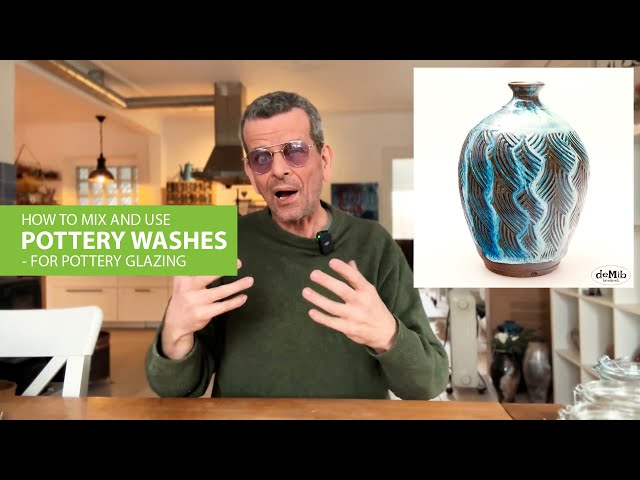This image appears to be a thumbnail or screengrab of a video tutorial on how to mix and use pottery washes for pottery glazing. The rectangular frame is horizontally oriented with narrow black letterbox bars at the top and bottom. At the center, there is a photograph of a man, a white older individual with short, salt-and-pepper hair and a beard, wearing a grayish-green sweatshirt. He has tinted glasses and a lapel microphone with a green light attached to his collar. The man, visible from the waist up, is seated at a light brown wooden table and is gesturing with his hands as he talks, likely into the camera. On the left side of the image, there is a green rectangle with white text that reads: "How to Mix and Use Pottery Washes for Pottery Glazing." To the right of the man, imposed on the image, is a white square background featuring a detailed blue and brown vase. In the background, elements of what appears to be a pottery studio can be seen, including some pottery pieces on the ground, a large silver metal vent hood, and a hanging light fixture. The setting and the man's focus suggest an instructional environment, geared towards demonstrating pottery techniques.